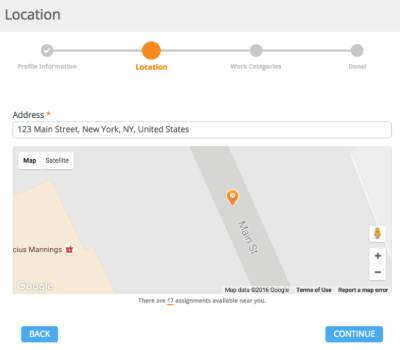A screenshot of a mobile phone display showing a sequence of steps in a process. At the top, there is a header with the word "Location," immediately followed by "Profile Information," both connected by a faint gray line. A series of icons along this line indicate various steps: a white checkmark within a gray circle represents a completed step, connected to the orange-highlighted "Location" step, suggesting the current focus. An orange circle above the word "Location" and the word itself in orange stand out, emphasizing the active step.

Continuing right, the gray line extends to another gray circle labeled "Work Categories," and finally to another gray circle that reads "Done," marked with an exclamation point. Below this sequence, the address "123 Main Street, New York, NY, United States" is displayed with an orange star beside it for further emphasis.

The bottom section features a map centered on Main Street, marked with an orange pin. Options to view the map in standard or satellite modes are present. At the very bottom, navigation buttons in blue provide a means to interact: a "Back" button on the left and a "Continue" button on the right.